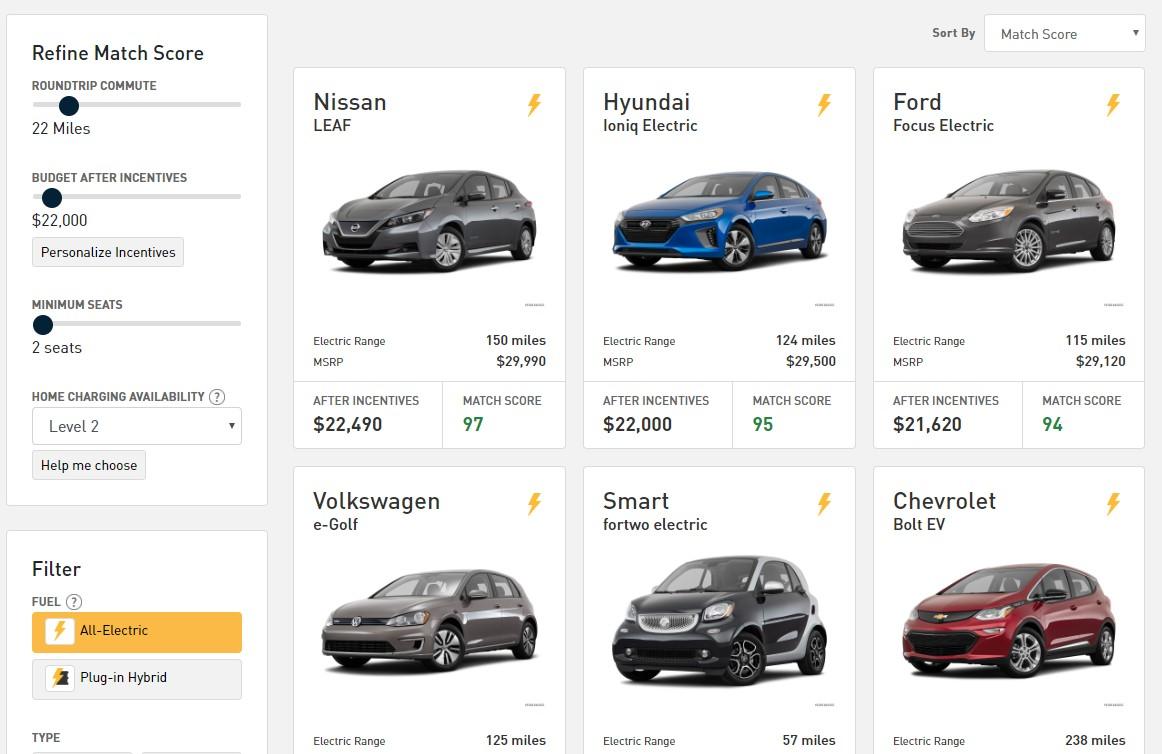The webpage offers a selection of cars for sale, conveniently allowing users to refine their search with detailed filters. On the left, a panel invites users to adjust their match criteria by specifying their commute distance, budget after incentives, desired number of seats, and home charging availability. In this example, the filters are set to a 22-mile round trip commute, a budget of $22,000, at least two seats, and access to home charging. Below these options, another filter allows users to select their preferred type of fuel, such as all-electric or plug-in hybrid.

To the right of the filters are six boxed options, each presenting a different car model. The options include:

1. **Nissan Leaf**: Priced at $22,490 with a 97% match score, offering an electric range of 150 miles.
2. **Hyundai Ioniq Electric**: A blue car listed at $22,000 with a 95% match score and an electric range of 124 miles.
3. **Ford Focus Electric**: A gray model costing $21,620, with a 94% match score and an electric range of 115 miles.
4. **Volkswagen E-Golf**: This model provides an electric range of 125 miles, although its price and match score are not visible.
5. **Smart Fortwo Electric**: A small black car with a seating capacity of two, offering an electric range of 57 miles.
6. **Chevy Bolt EV**: A red car with a substantial electric range of 238 miles, with the price and match score not displayed.

Each car listing includes details about the vehicle's electric range, aiding potential buyers in making an informed decision.